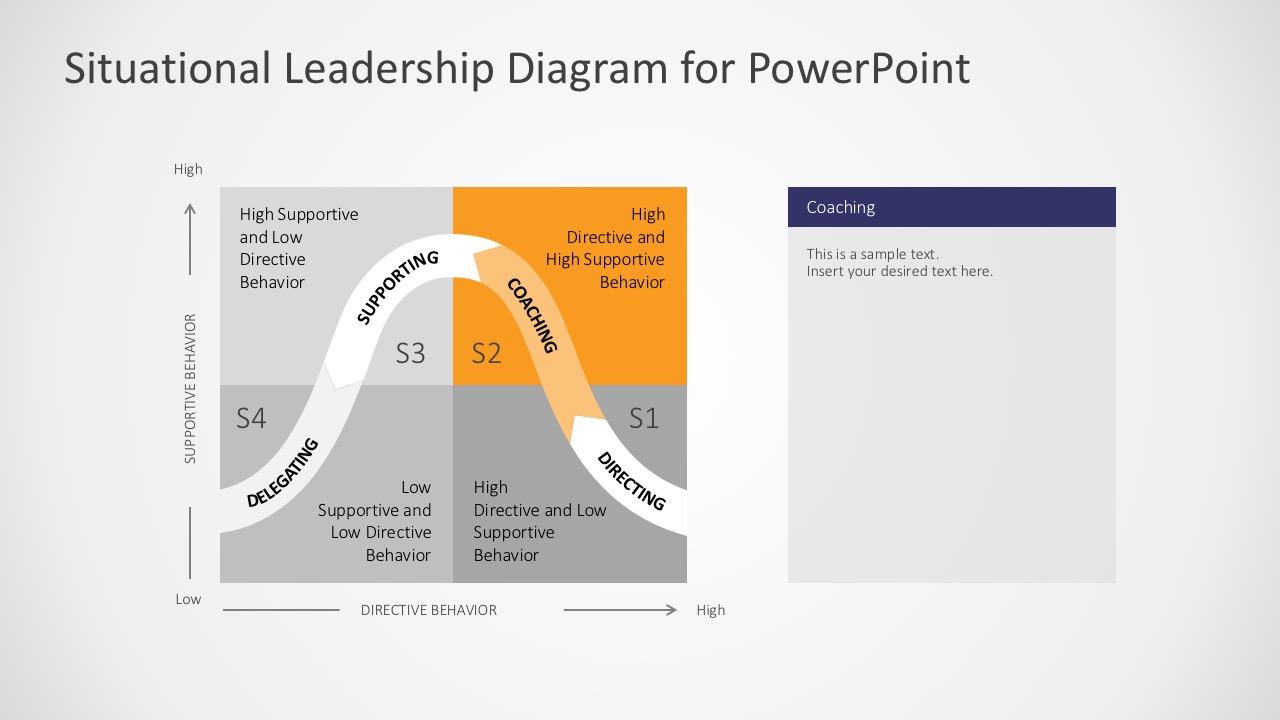The PowerPoint slide titled "Situational Leadership Diagram for PowerPoint" features a gray background with a detailed X over Y graph at its center. The Y-axis represents supportive behavior increasing from low to high, and the X-axis represents directive behavior increasing from low to high. The chart is divided into four colored quadrants: the bottom left is low supportive and low directive (S4, in light gray), the upper left is high supportive and low directive (S3, in a slightly lighter gray), the upper right is high directive and high supportive (S2, in orange), and the bottom right is high directive and low supportive (S1, in dark gray).

An arc or curve overlays these quadrants, starting at the bottom right with 'Directing' (S1), peaking at the top right with 'Coaching' (S2), slightly descending to the top left with 'Supporting' (S3), and ending at the bottom left with 'Delegating' (S4). The curve visualizes the shift in leadership styles over different levels of supportive and directive behavior. Each quadrant label emphasizes the contrast between directive and supportive behaviors, showcasing where each leadership style fits within the situational context. Customizable text boxes are present, allowing for further annotations or examples.